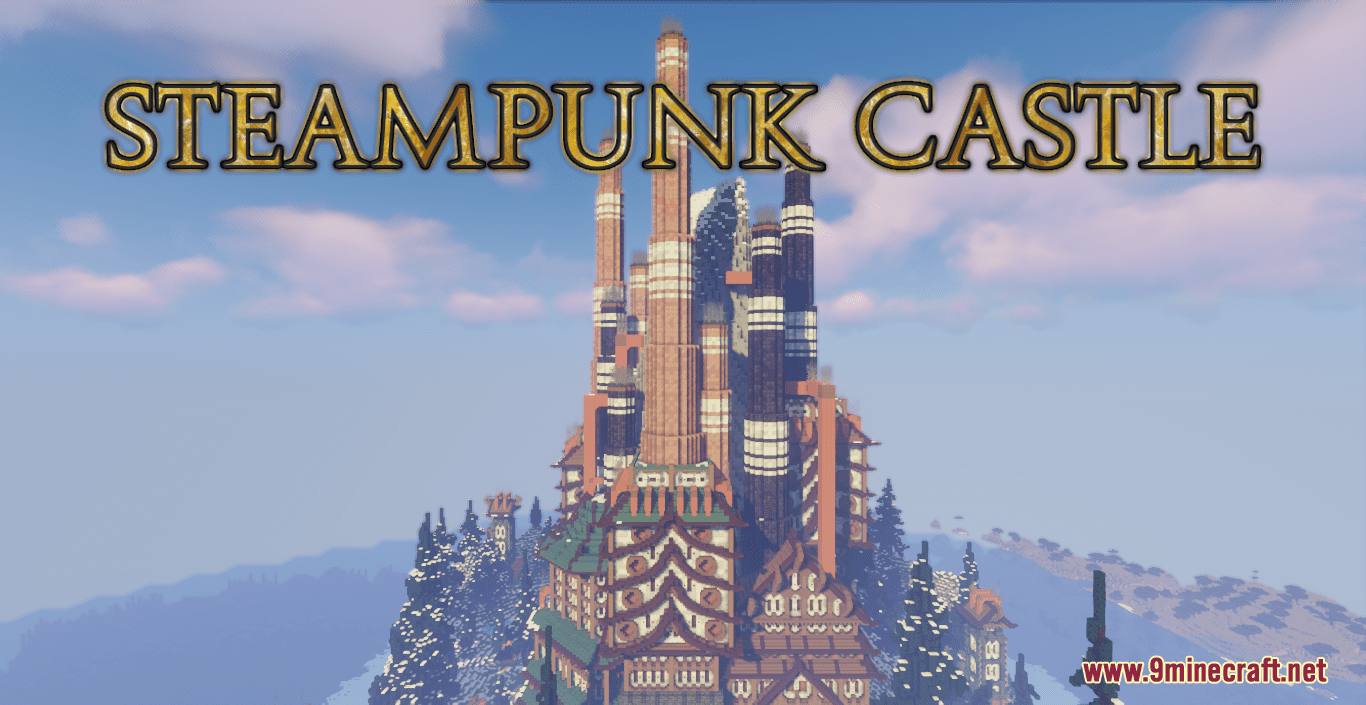The image, set in a horizontal rectangle, features a striking digital art depiction of a steampunk castle centrally positioned. This fairytale-like castle is adorned with multiple towers of varying heights and colors such as brown, black, and purple, each accented with distinctive white stripes. The architectural style suggests a blend of toy-like whimsy and Bavarian influences, complete with cylindrical-shaped structures and sections resembling regular buildings with V-shaped roofs.

The background consists of a serene blue sky dotted with white and grayish clouds, enhancing the castle's ethereal quality. At the top of the image, the title "Steampunk Castle" is prominently displayed in gold letters with a black outline, stretching from left to right across the castle scene. In the bottom right corner, the text “www.9minecraft.net” appears in small red letters, indicating the origin of the image from a Minecraft-related website.

Surrounding the castle are lush evergreen trees, and the landscape includes hills that descend and rise on either side of the castle, adding depth and a picturesque setting to the composition.